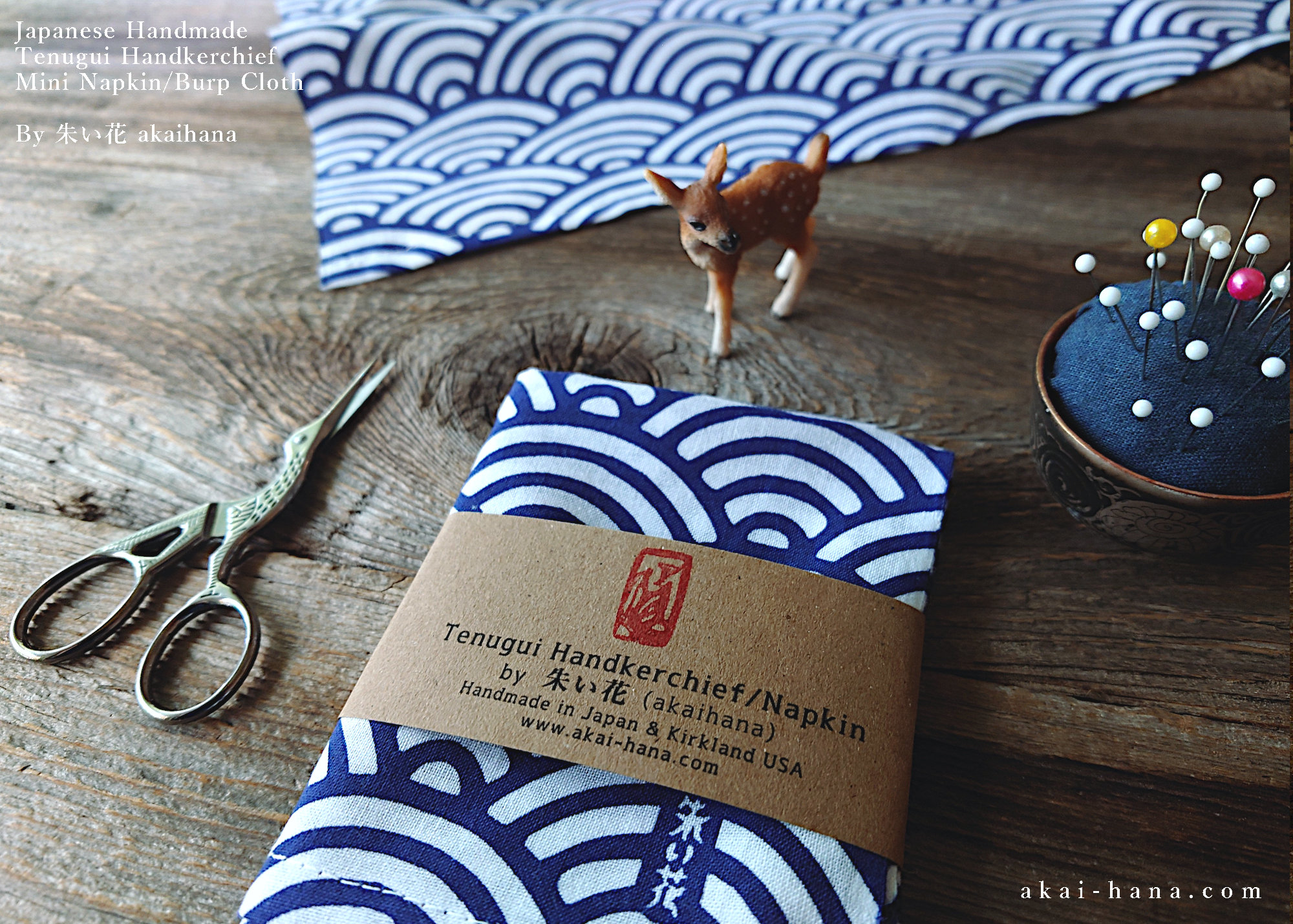The image features a close-up view of a product display on a brown wooden table, showcasing a meticulously folded Japanese handmade Tenugui handkerchief by Akai Hana. The handkerchief, adorned with a sophisticated blue and white wave pattern resembling concentric circles, is wrapped with a brown cardboard band featuring a red company logo stamp and the text "Tenugui handkerchief/nakpin by Akai Hana, handmade in Japan, in Kirkland, USA, www.akai-hana.com."

To the top of the image, another sample of the handkerchief is laid out, displaying its decorative design. Central to the scene is a whimsical and realistic-looking miniature toy deer, adding a playful touch. Surrounding the handkerchief is a brass pair of bird-shaped scissors and a needle holder filled with sewing pins—white ball-headed with a few pink and yellow ones—highlighting the handmade nature of the product. Additionally, the top left corner of the image contains text reading "Japanese Handmade Tenugui Handkerchief and Mini Napkin/Burp Cloth by Akaihana," along with a simple, patterned blue and white tablecloth crafted by a Japanese company.